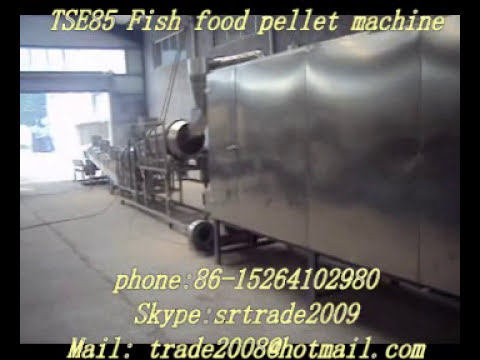The image depicts the interior of an industrial building, featuring a large and sophisticated piece of equipment labeled "TSE 85 Fish Food Pellet Machine" in light yellow text at the top. The bottom of the image displays three lines of similarly colored text, providing contact information: a phone number (86-1526410298), a Skype username (SRTRADE2009), and an email address (Trade2008 at Hotmail.com). The machine, primarily constructed from gray metal with chrome elements, dominates the scene. It includes a series of intricate tubes and a conveyor belt system that stretches from a central stainless steel container towards an open garage door, allowing sunlight to pour into the otherwise concrete-floored space. The entire image is bordered by a black frame, emphasizing the detailed industrial setup within the garage-like environment.